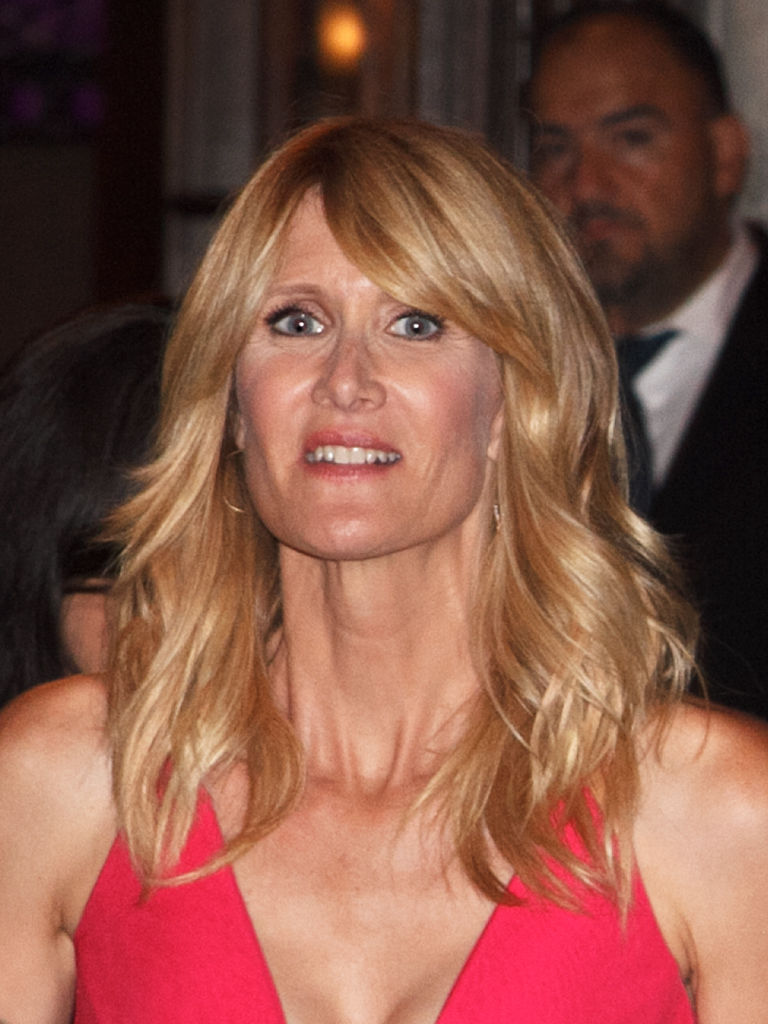This color portrait photograph features the actress Lara Dern, captured from her upper chest and above. She is wearing a sleeveless, low-cut, light red dress with a v-neck, and gold hoop earrings. Her long blonde hair, adorned with bangs in the front, cascades below her shoulders. Lara's lips are painted a reddish hue, and her mouth is partially open, revealing the top row of her teeth. She has striking green eyes that gazes forward, creating a captivating focal point. 

In the background, above Lara's top shoulder, is a man. He has a dark complexion and is dressed in a black business suit, a white shirt, and a black tie. His facial hair includes a dark mustache and beard. To the left, slightly above Lara's left shoulder, there is a partial view of the top of another person's head. 

The setting of the photograph is indoors, with light-colored curtains and a light source visible through a window in the background. The photographic style is representational realism, capturing minute details and elements with clarity and precision.